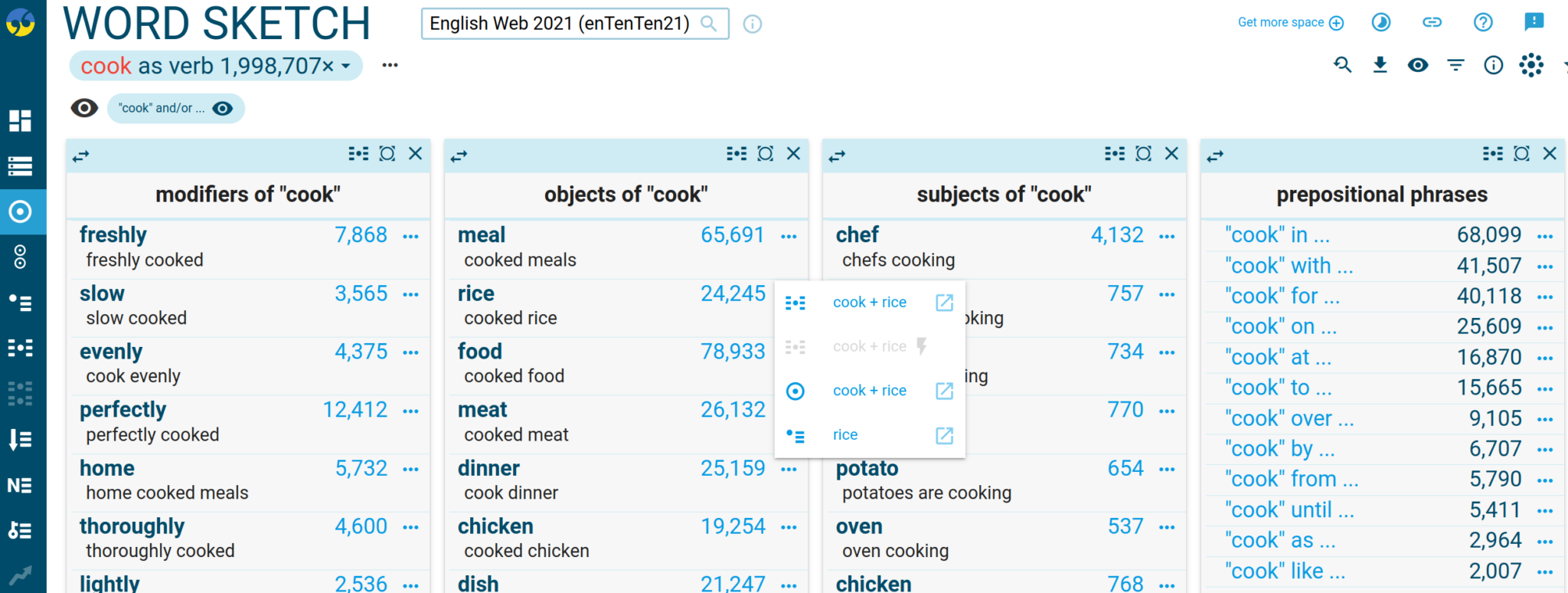This image is a screenshot of a computer application featuring a teal sidebar on the left side. At the top of the sidebar, there is a logo that consists of a circular design with a yellow bottom half and a blue top half. This logo also includes a teal comma in the bottom left corner and an inverted teal comma in the top right corner. Below the logo, there is a series of white icons:

1. The first icon is composed of white rectangles arranged in a square shape.
2. The second icon displays three horizontal white lines, each accompanied by a teal dot on the left side.
3. The third icon is a white circle surrounded by a light blue donut shape, which is further encircled by a white circle and then by a light blue square.
4. The fourth icon mirrors the third but features two smaller white circles stacked vertically.
5. The fifth icon shows three horizontal white lines in a vertical stack with a white dot to the left.
6. The sixth icon consists of three shorter vertical white lines stacked on the left and right sides, with a white dot in the middle.
7. The seventh icon is similar in layout to the sixth but uses medium blue color, with only two vertical lines in each stack.
8. The eighth icon displays three horizontal white lines stacked vertically on the right, accompanied by a white downward-pointing arrow to their left.
9. The final two icons are also white, accompanied by one additional medium blue icon, continuing the visual theme established above.

This detailed arrangement of icons contributes to the interface's visual hierarchy, aiding in the application's navigation and functionality.